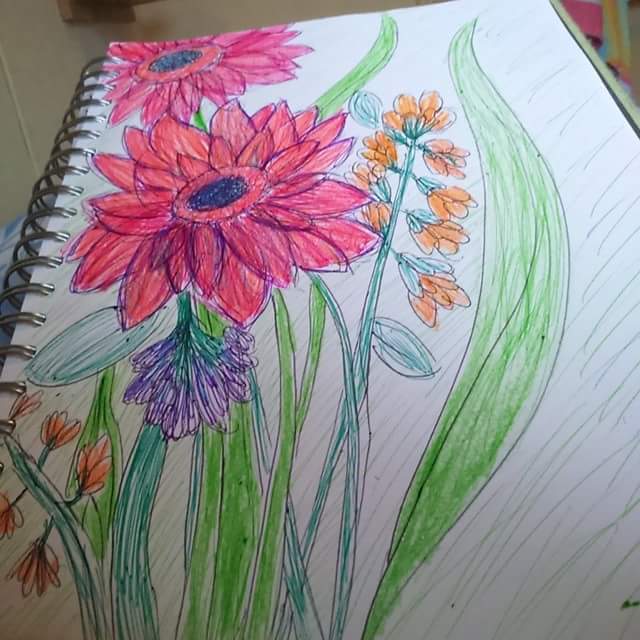This image features an intricate drawing of flowers and plants on a white sketchbook page. The sketchbook is bound with silver spirals on the left side, clearly visible in the photo. The background includes a white wall on the top left, while the top right showcases a blurry yet colorful element with shades of pink, yellow, and light blue. The focal point of the drawing is a prominent, large flower with vivid red petals. The flower's stems vary in color, with some shaded in green and others in teal, adding depth and variety to the botanical artwork.